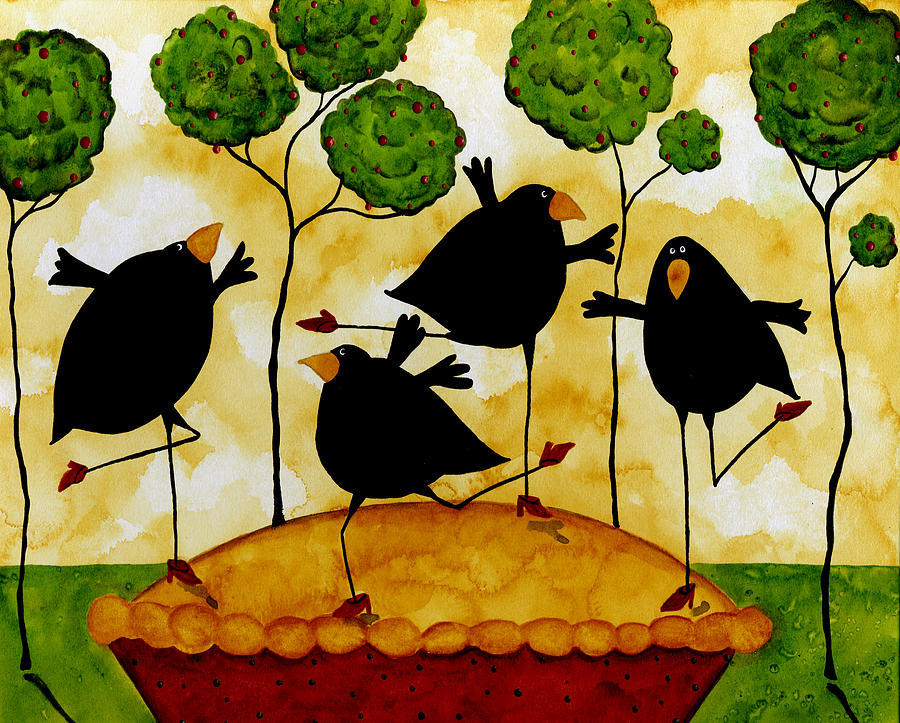This vibrant and eclectic painting by Nathalie Scherr features a whimsical scene brimming with vivid colors and playful details. At the center of the artwork, four black crows with yellow beaks and very long legs are depicted dancing in a circular motion atop a generously oversized baked pie, which rests in a striking red pie dish. The crows, each sporting red high heels, add a humorous twist to the scene as they prance around the golden-brown, freshly baked pie. Surrounding this comedic centerpiece, a backdrop of green grass is punctuated by four trees. Each tree has a thin trunk and a circular canopy of leaves, adorned with numerous red berries or fruits, likely apples. Completing the ensemble, a splotchy yellow watercolor background adds to the abstract and whimsical charm, making this piece a delightful fusion of surreal and playful elements.